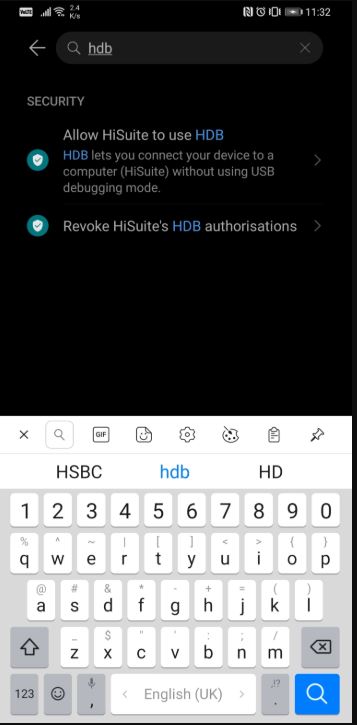This image is a screenshot taken from a smartphone. The background of the image at the very top is black, transitioning to white toward the bottom where a virtual QWERTY keyboard is visible. The keyboard features white keys with gray letters and numbers, and some functional keys at the bottom are in gray as well. The space bar remains white.

At the very top of the keyboard, there are text elements: "HSBC" is presented at the top, followed by "HDB" in blue, and then "HD" in gray. 

Moving to the upper half of the image, there is a search box with a light gray color against the black background, displaying "HDB" in light gray font. Below the search box, in gray font, the text reads "security" followed by "allow HiSuite (H-I-S-U-I-T-E) to use." The abbreviation "HDB" is highlighted in blue font within the same line. 

Directly beneath this, a description in gray font clarifies: "HDB lets your device connect to a computer, using HiSuite, without enabling USB debugging mode." Lastly, at the bottom of this section, the text "revoke HiSuite's HDB authorizations" is presented in white font.